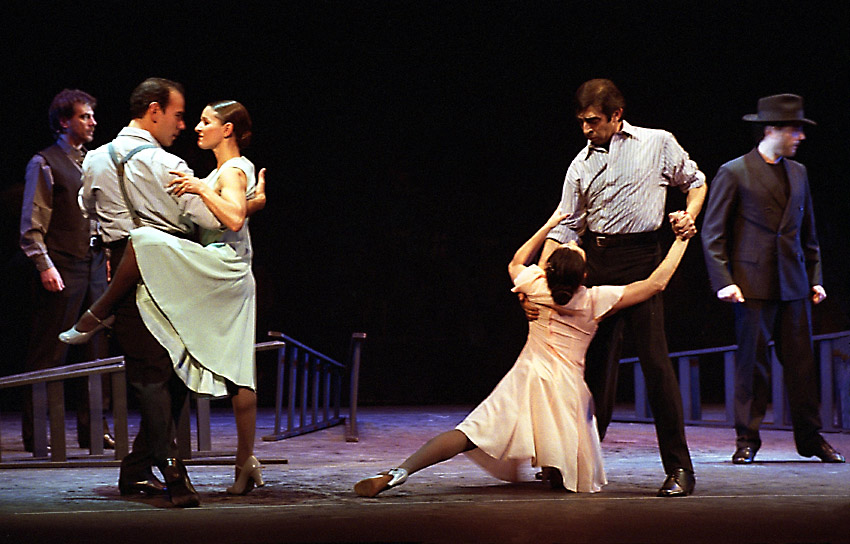This full-color photograph, taken indoors during a play, features six performers on a stage with a completely black background. The theatrical scene is vividly captured with four men and two women, each engaged in dramatic or dance poses. 

On the far left, a man with black hair, wearing a light-colored gray shirt, a dark vest, and dark pants faces slightly forward to the right. Next to him, closer to the foreground, another couple captivates the viewer’s attention. The man, wearing a light-colored shirt and dark pants, is observed from behind, his head turned rightward as he looks at his dance partner. This woman, ensconced in a blue dress, wraps her left leg around his waist, balancing on her right foot. Her medium-length dark hair flows as she gazes at him, embodying the essence of their dance.

Scattered between these figures are ladders laid on their sides, adding a touch of backstage authenticity to the staged scene. 

To the right of the center, another dancing couple commands attention. The woman, dressed in a peach-colored dress, kneels with her left leg swept behind her and looks up at her partner. Her left arm reaches towards his right, while her right hand rests in his left. The man, with short dark hair, wears a light shirt and dark pants. He stands facing forward but looks down at her, maintaining a connection that speaks of tenderness and choreography.

On the far right, a solitary man stands, donning a black suit and hat but no tie. His body faces forward, yet his head is turned to the right, mirroring the posture of the man on the far left. This positioning creates a frame around the central dancers, focusing the audience’s gaze on the dynamic interplay between the performers.